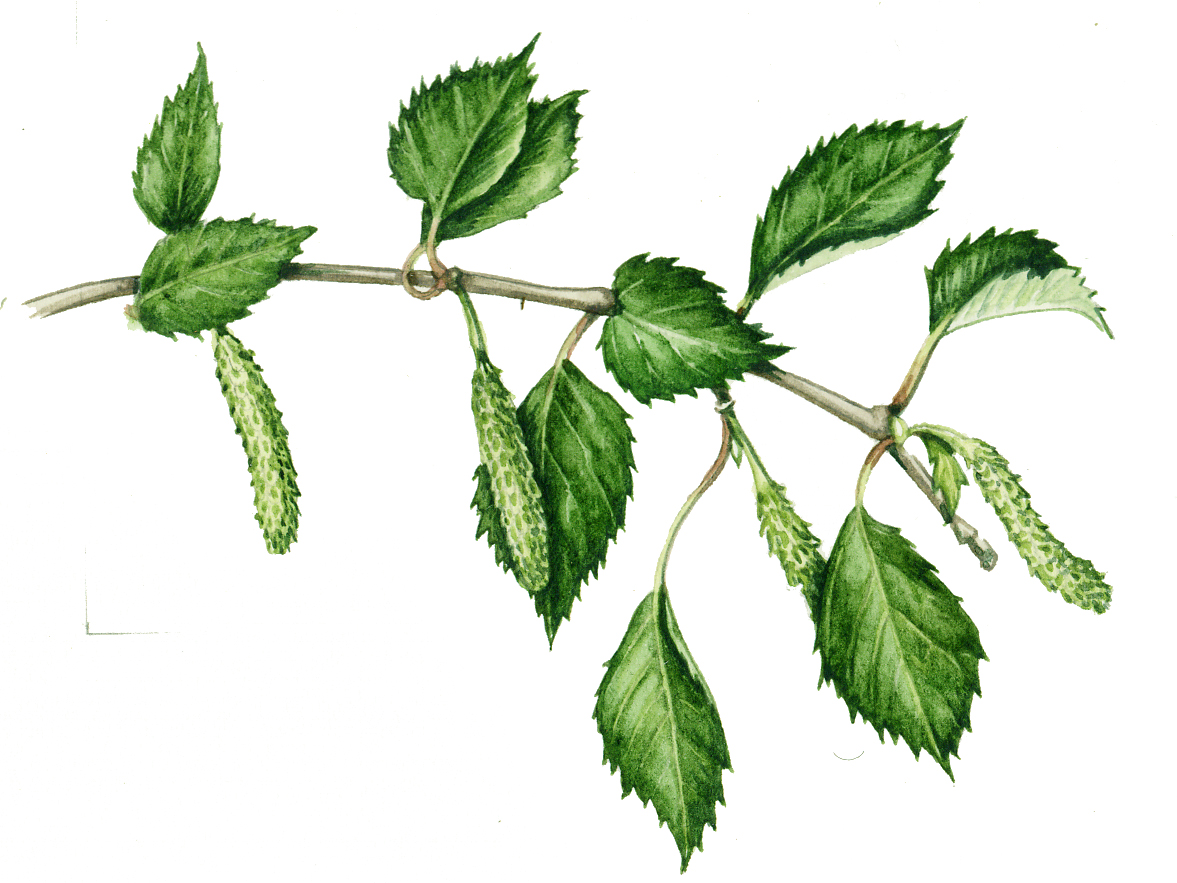The image presents a detailed drawing of a branch against a white background, extending from the left center down to the right bottom, curving slightly downward. The branch, depicted in a subtle grayish tone, is adorned with multiple green leaves. Strikingly, there are four elongated, green, bumpy structures hanging from the branch, which resemble small cucumbers or cocoons, with a slightly lighter green hue than the leaves. These peculiar structures give the impression of being either the plant's early fruiting bodies or seed pods, or even something akin to cocoons or chrysalises, suggesting a close interaction with nature’s lifecycle. The drawing captures the delicate balance of the branch with its various elements, creating a sense of natural growth and development.